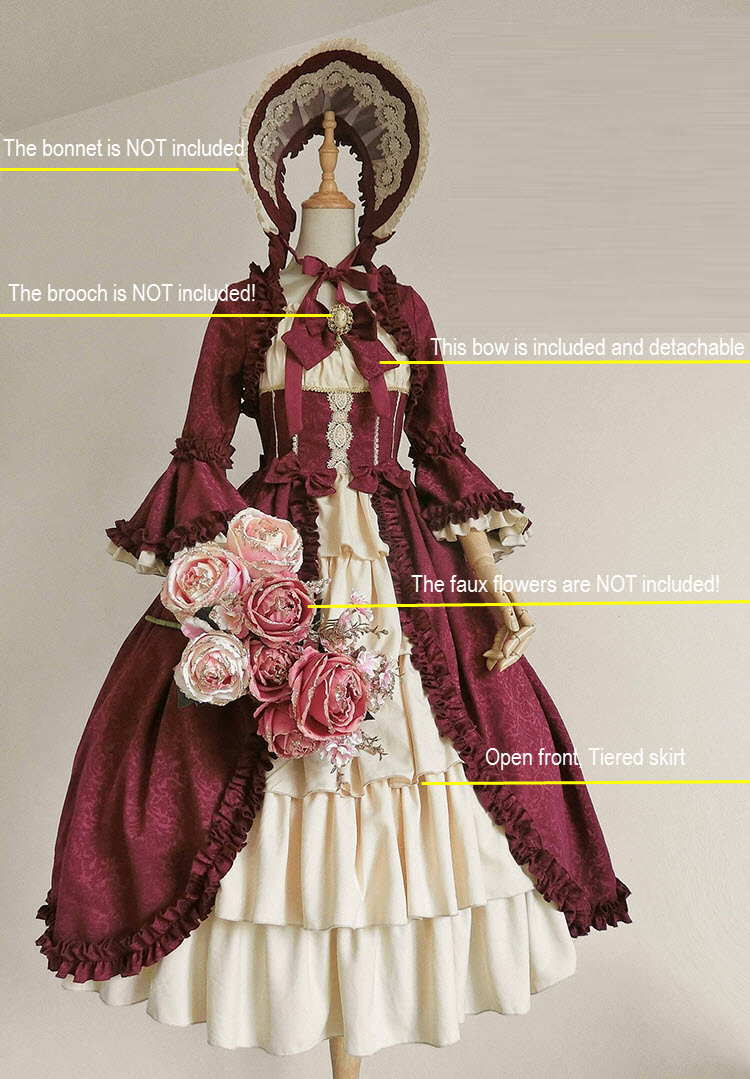This advertisement photograph features a headless mannequin displaying a Victorian-style dress, characterized by its intricate, multi-layered design. Atop the mannequin is a bonnet held by a peg, which is white and red; however, a note specifies that the bonnet is not included. The dress features a ruffled white petticoat beneath an overlay of red and white brocade or damask fabric. The bodice includes a red corset accented by a detachable bow, and there's a brooch near the neckline, although the brooch itself is not included. The mannequin's hand holds a bouquet of faux flowers in shades of pink and red, which are also not included. Additional text notes describe the dress's features, such as the open front tiered skirt. The overall design and elements of the dress suggest it hails from the late 1800s to early 1900s, evoking a distinctly old-fashioned, Victorian elegance.